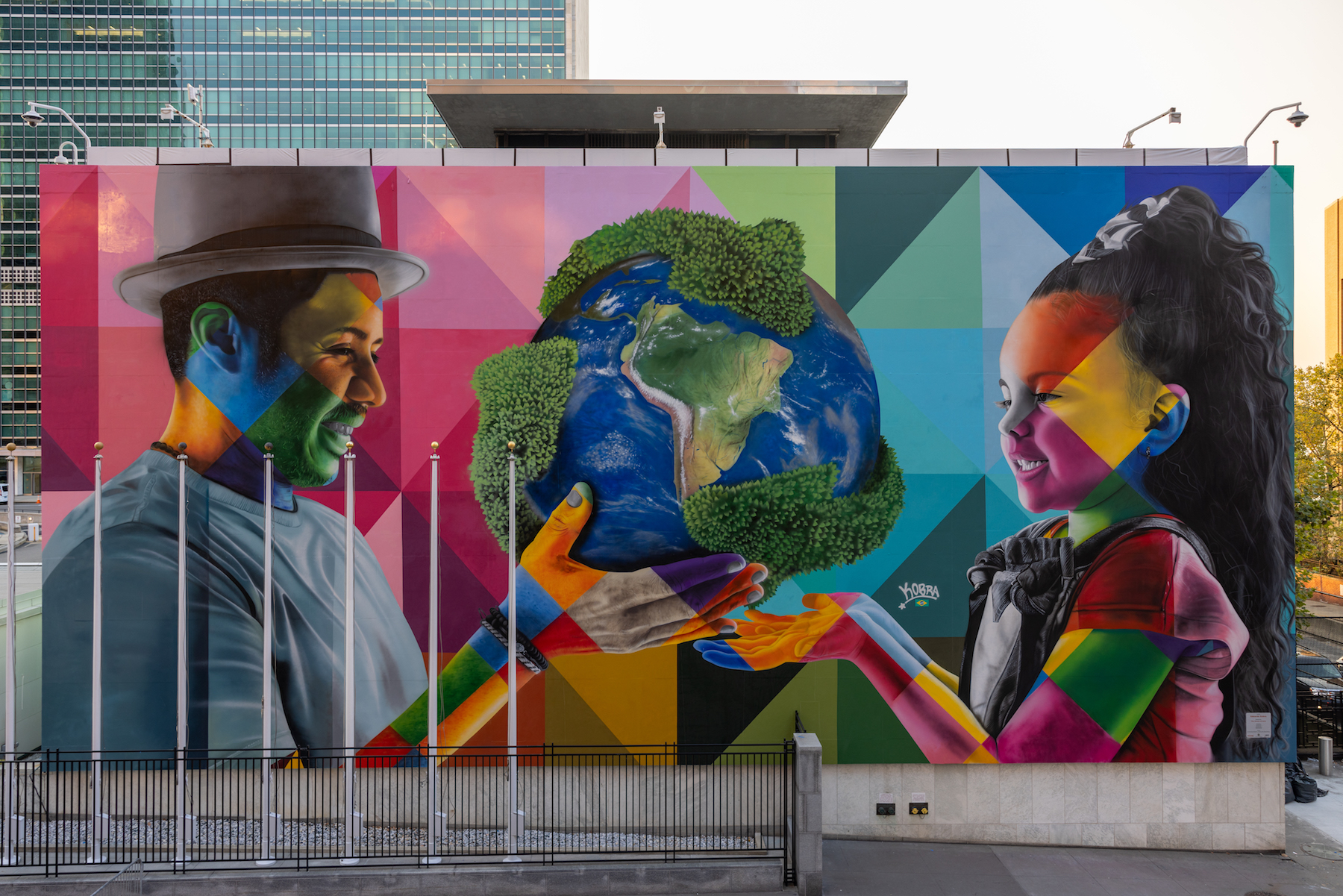The photograph captures a vibrant and captivating mural spread across the side of a large building, which is further accentuated by the daylight illuminating it and by five lights positioned at the top. The mural, likely 40 feet tall and 60 feet wide, uses a mosaic of colors and grayscale tones arranged in a kaleidoscopic pattern of triangles and checkerboard squares, seamlessly blending reds, pinks, greens, yellows, and blues. In the heart of the mural, an African-American man, possibly around 40 years old and wearing a gray bowler hat, stands on the left. He is holding a caricature of the Earth, depicted as a large beach ball-sized globe adorned with green grassy patches and sprouting vegetation. He appears to be handing it to a young African-American girl, perhaps seven or eight years old, on the right. She has long, thick curly hair, a bow, and outstretched hands ready to receive the globe. Beneath the mural, a stone wall supports part of the structure, and a metal and concrete fence can be seen along the lower left half. Behind the mural, a large building with several glass windows and a glimpse of the sky in the upper right corner adds depth to the background. The entire mural symbolizes the man's willingness to give the world to the young girl, encapsulated in a scene bursting with color and life.